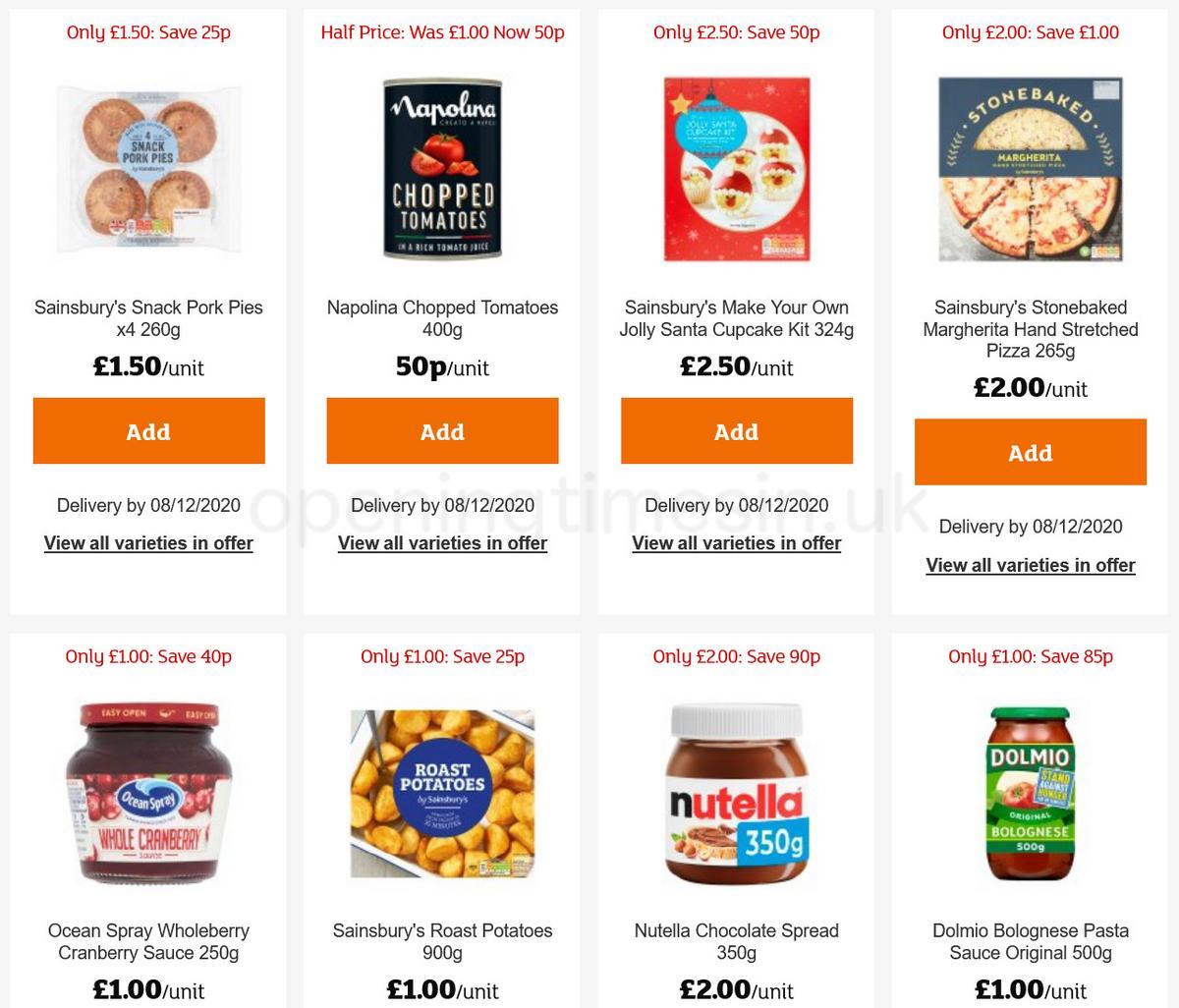This image is a screen capture of a webpage from an online grocery store, showcasing a selection of available grocery items arranged in two rows, each containing four products. The top row features the following items:

1. Sainsbury's Snack Pork Pies
2. Napolina Chopped Tomatoes
3. Sainsbury's Make Your Own Jolly Santa Cupcake Kit
4. Sainsbury's Stone-Baked Margarita Hand-Stretched Pizza

The second row includes:

1. Ocean Spray Whole Berry Cranberry Sauce
2. Sainsbury's Roast Potatoes
3. Nutella Chocolate Spread
4. Dolmio Bolognese Pasta Sauce, Original

Each product tile presents a detailed view, featuring:

- A clear and colorful picture of the item.
- The name of the product prominently displayed.
- The price of the item and any applicable savings or sale price.
- The weight of the item in grams.
- An orange "Add" button, allowing users to add the item to their shopping cart.
- A delivery date.
- An option to "View All Varieties" at the bottom of each tile, enabling users to explore other available options.

The layout is designed for ease of use, with each product image accurately representing its appearance upon delivery.